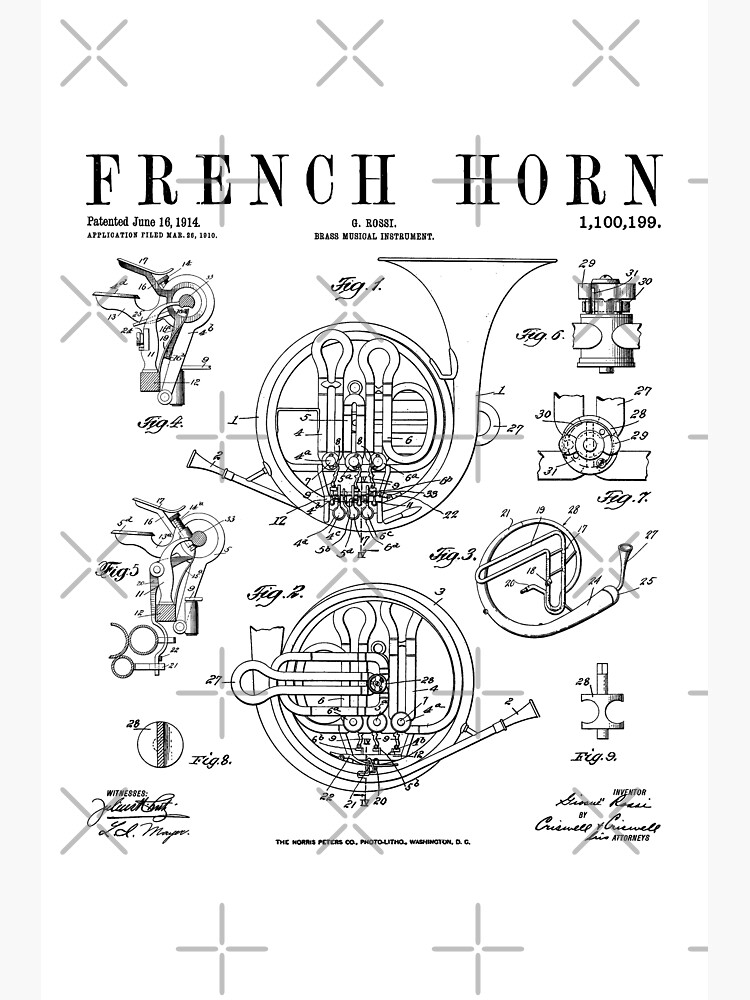The black-and-white image is a detailed patent diagram of a French horn, dated June 16, 1914, under the heading "French horn" at the top. The left side of the page bears the patent date, while to the right, it states "G. Rossi Brass Musical Instrument" alongside the patent number 1,100,199. The image features multiple intricate diagrams labeled "fig 1," "fig 2," etc., showcasing various parts and mechanical details of the French horn. Scattered across the page are crosshairs, with gaps in their intersections, framing the technical illustrations. In the bottom corner, difficult-to-read small text includes "Washington, D.C."